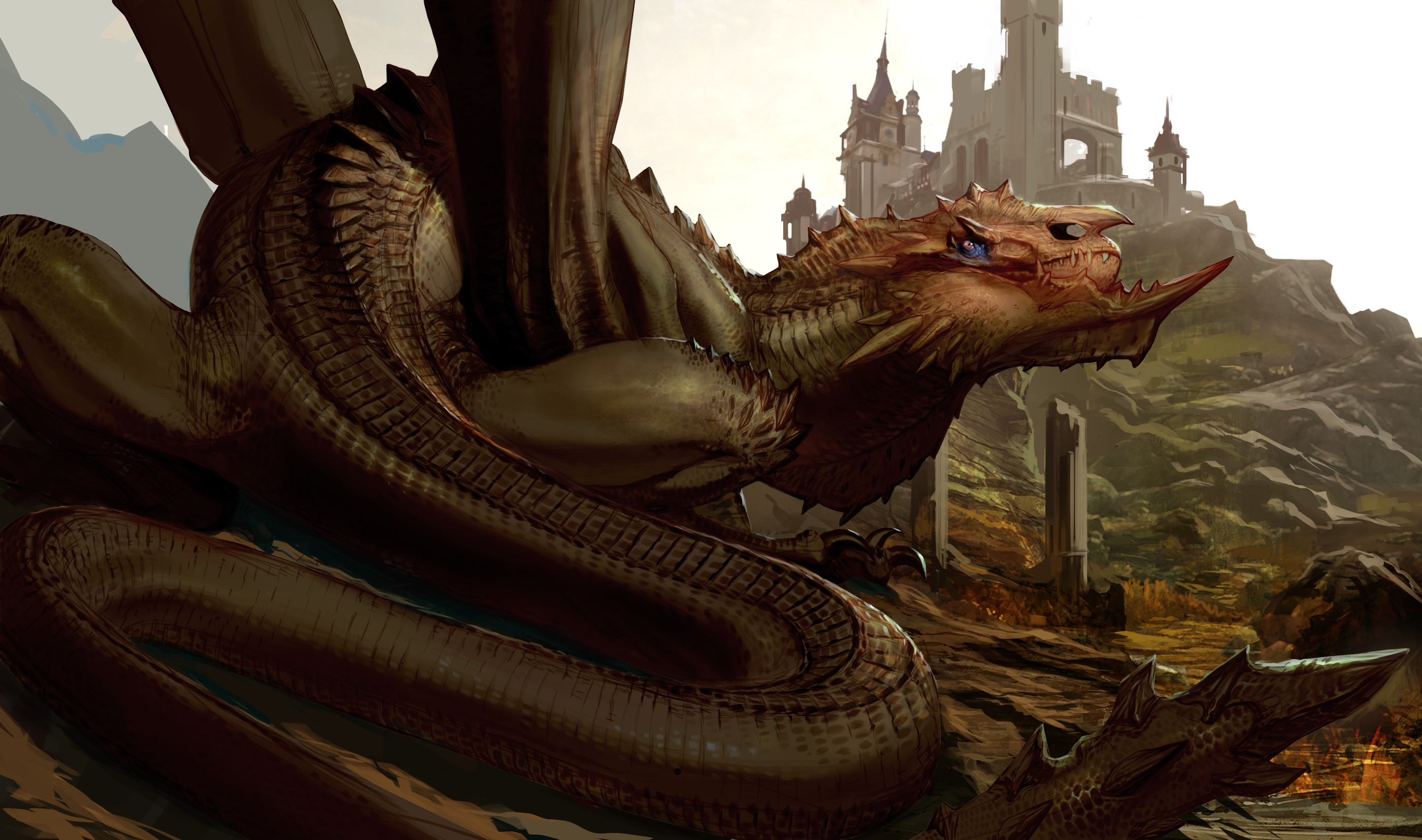A captivating artwork by a talented graphic artist depicts an enchanting scene during the day. Dominating the background, a grand medieval castle rests atop a hill, its majestic grey towers tinged with hints of brown. The cloudy sky forms a nearly white canvas, adding an ethereal quality, while distant mountains peek through on the far left, creating a sense of vastness.

The castle itself is surrounded by patches of verdant grass, and intricately designed columns are faintly visible, suggesting an architectural marvel perched on rugged terrain. In stark contrast to the serene backdrop, the foreground features a formidable brown dragon occupying the scene with its imposing presence. The dragon’s long wings are partially out of view, and its sinuous tail curls artfully around, with only segments visible. Along the top of its body, ridges resembling scaled claws add to its menacing appearance.

The dragon’s face, a lighter brown with an orange hue, is adorned with striking blue eyes, and a subtle streak of blue underlies its form. Its tail, prominently displayed on the right, tapers into a sharp, dagger-like tip with jagged edges, clearly designed for a fierce defense. Dark, menacing black claws dig into the ground, hinting at its readiness to strike.

With its mouth closed, the dragon appears calm yet vigilant, surveying its domain with an air of regal authority. This detailed and vivid scene masterfully combines elements of fantasy and realism, drawing viewers into a mythical world where dragons and castles coexist.